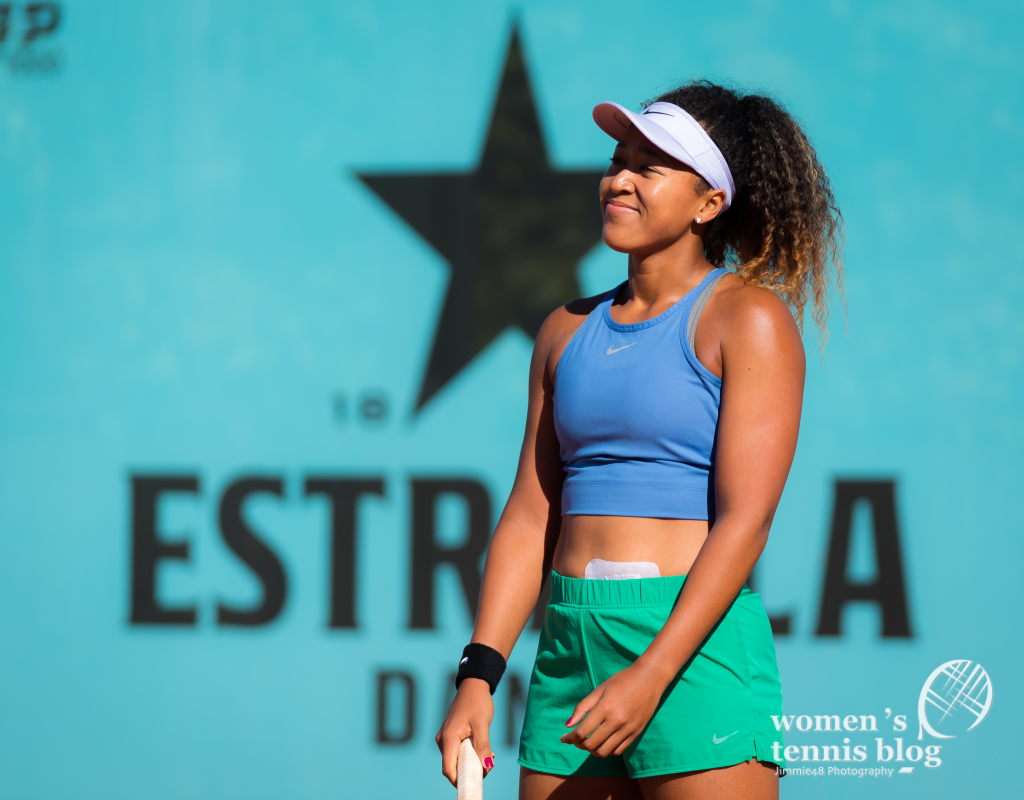The photograph depicts an African-American female tennis player with long, wavy brown hair that has red and blonde tips. She is beaming a bright smile and wearing a white Nike visor along with a blue Nike sports tank top that reveals her midriff. Adorning her right wrist is a black sweatband, and she holds a white tennis racket in her right hand. She is dressed in green shorts with a bandage visibly placed above them. The photo features a logo in the bottom right corner that reads "Women's Tennis Blog" accompanied by a racket graphic. Behind her is a background that appears blue and has a partial word with a black star, likely "ESTR" or "a strata," though her figure obscures the complete text.